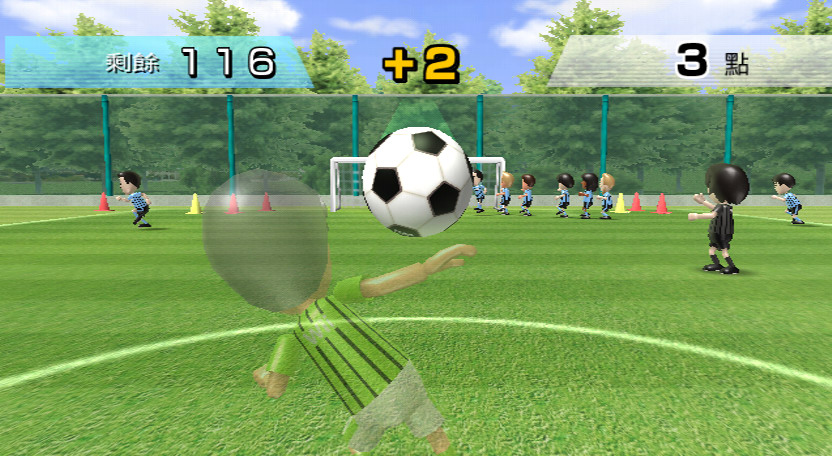This horizontally oriented screen capture depicts an animated soccer game reminiscent of a Wii sports game with an Oriental theme. The scoreboard at the top of the screen shows a current score of 116 for one team and 3 for the other, with a prominent yellow "+2" symbol displayed at the center. The soccer ball is in mid-air, positioned just slightly above the center of the image. In a dynamic action pose, a semi-transparent player in a green jersey and white shorts appears to be preparing to head the ball. In the background, a line of players in blue uniforms is strategically positioned near the goal net. A referee dressed in black stands off to the right center of the frame. The setting features a lush green playing field with trees and a high fence visible in the distance, running horizontally across the image.